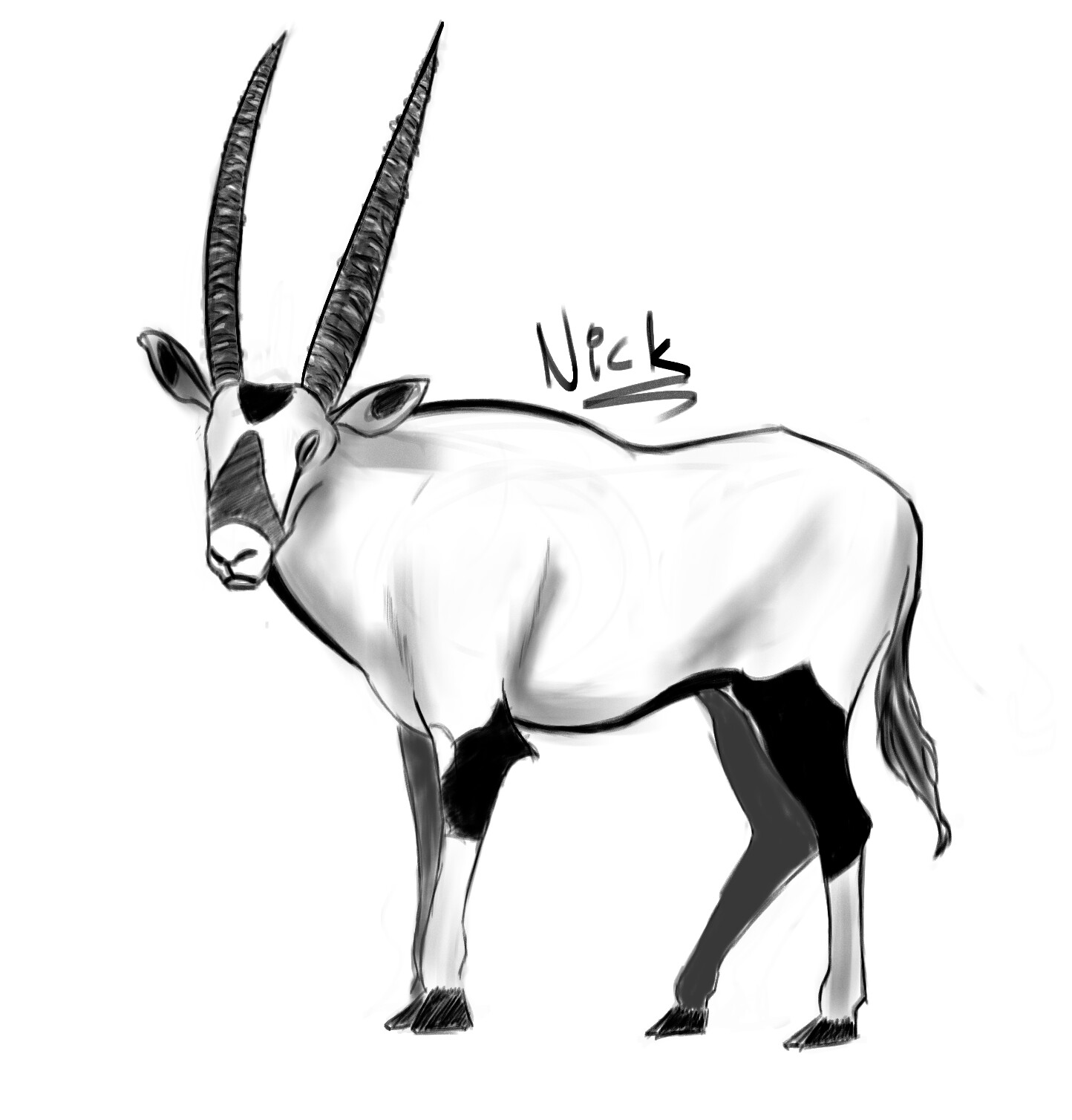The image is a detailed, hand-drawn line illustration of an African antelope-like animal, possibly a gemsbok or springbok, rendered with markers on a white background. The animal is primarily black and white with shades of gray for shading. It is oriented facing the left side, standing on all four legs, with its head turned slightly toward the viewer. The animal features strikingly long, sharp black horns that extend almost to the full length of its body, pointing straight up or slightly back without curving. Its face is predominantly white with patches of black on the forehead, top of the nose, and around the eyes, complemented by protruding ears. The body shows a mix of white with black markings on the upper thighs and black hooves. Above the animal, on the blank background, the artist has signed the name "Nick," underlined by a squiggly line.